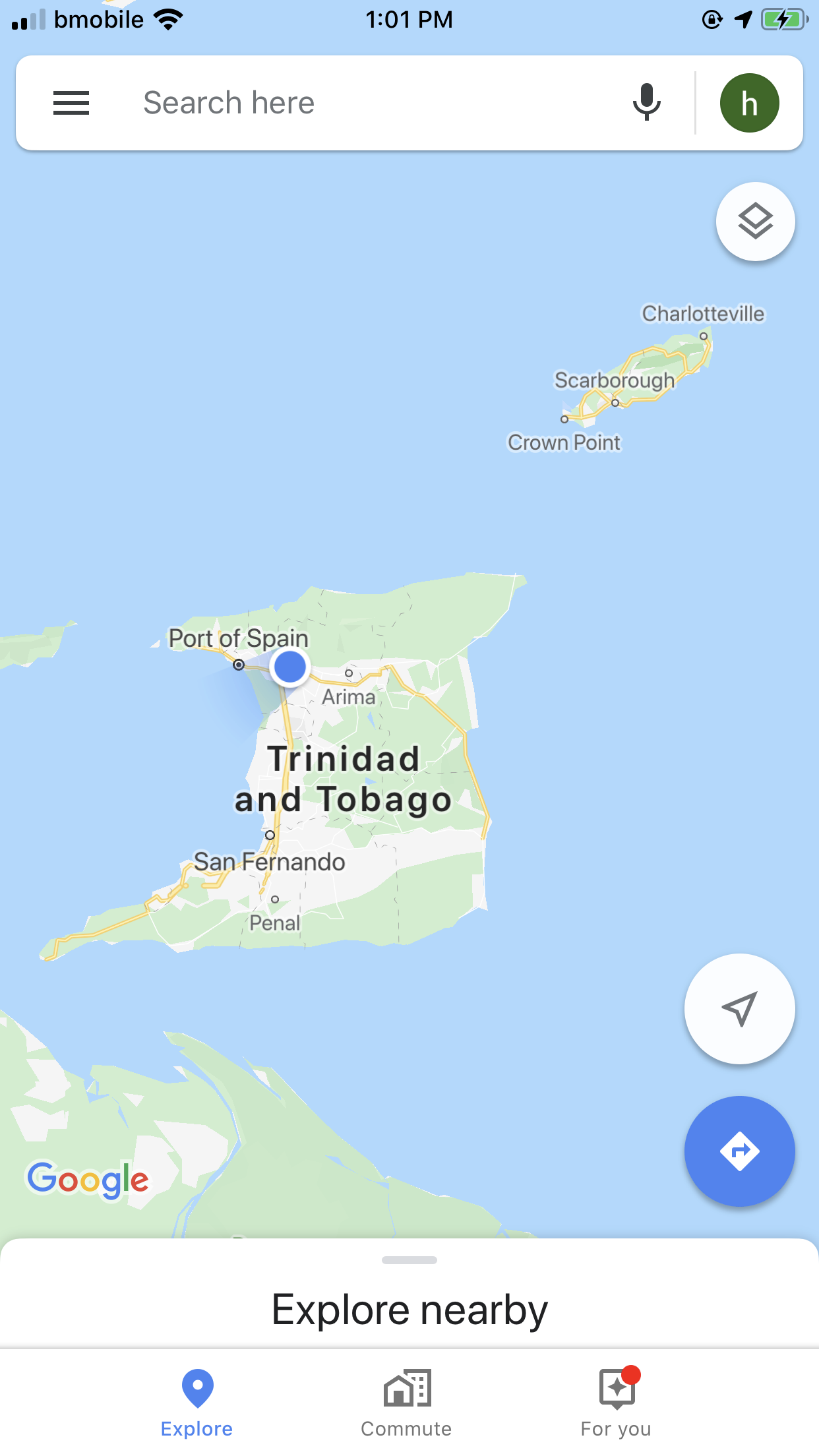Screenshot of a blue-background mobile interface from B-Mobile at 1:01 PM, with a full battery indicator. At the top, there's a search bar displaying "Search here" alongside a hamburger menu icon and a microphone icon. Below, a green circle with a white "H" is visible. Further down, a white circle contains two overlapping squares, representing a map. The map shows Trinidad and Tobago, with a prominent blue circle. At the bottom, a navigation icon is embedded in a circular element. Adjacent to this, a blue circle contains a white diamond with an upward right-pointing blue arrow, labeled "Explore Nearby." The screen also features options like "Explore," highlighted in blue, "Commute," and "For You." A small red circle appears at the top of the interface.